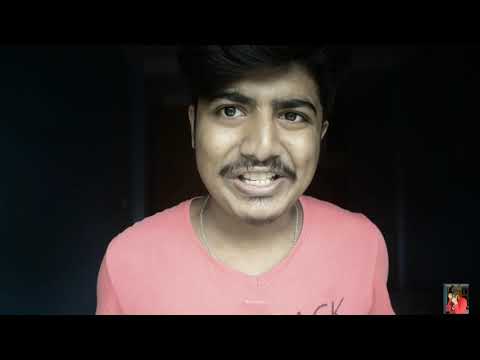A man, likely Hispanic, appears in a video call or streaming session, illuminated by his screen against a completely black background. His expression is neutral, with his mouth open mid-sentence, possibly explaining something passionately. He has brown skin, black hair parted to the left with wisps falling over his forehead, and brown eyes, with his right eye slightly squinted. He sports a mustache and a small goatee, and wears a salmon-colored shirt featuring the top parts of the letters "C" and "K," along with a small icon of a face with a white face and a red bow around its neck. Around his neck, he wears a necklace. In the bottom right corner of the screen, there is a small thumbnail of another person, possibly interacting with him. The image suggests he is engaged in a virtual conversation, perhaps reacting to something being shown by the person in the thumbnail.